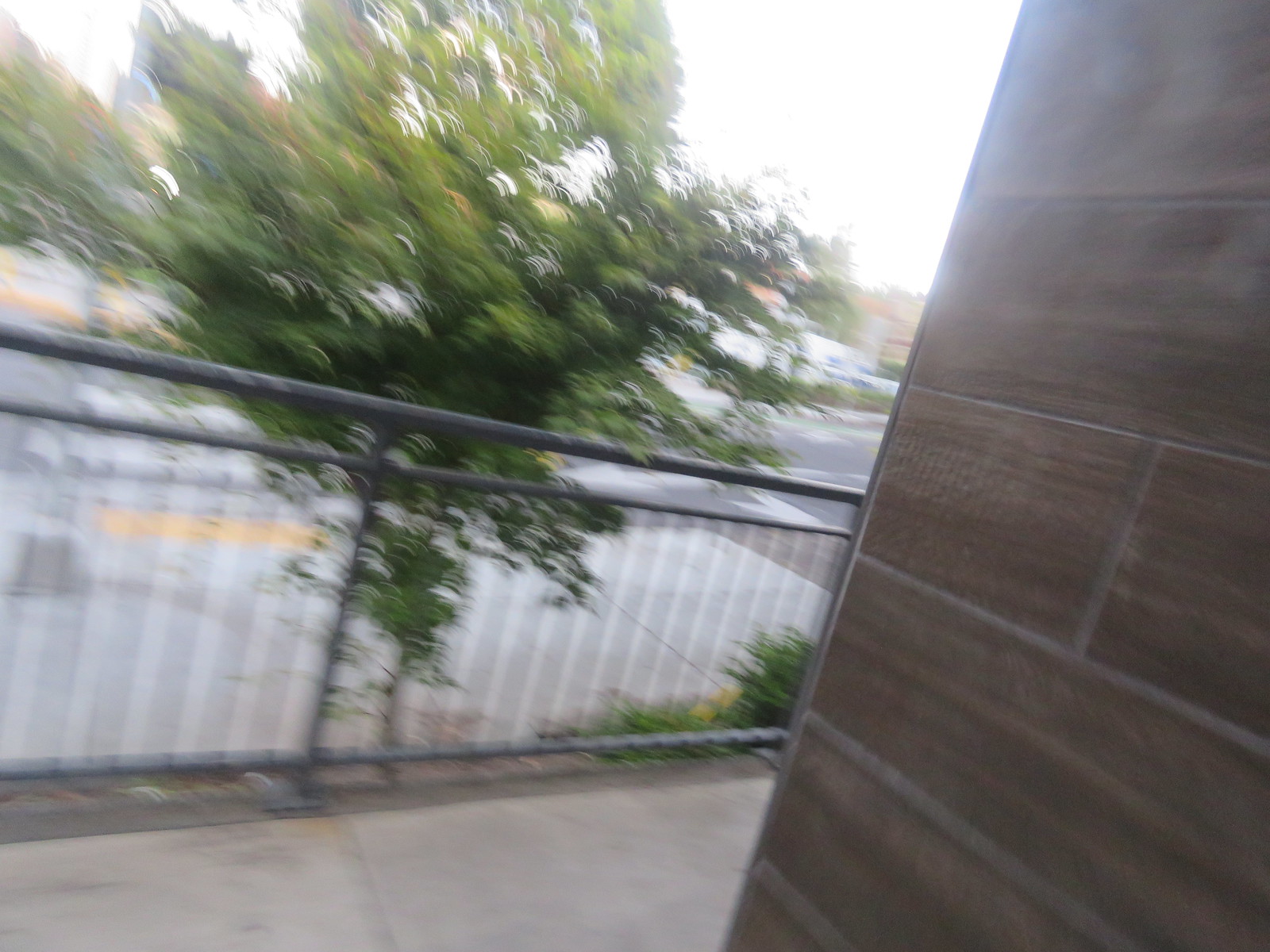The image depicts the corner of a brown brick building with light gray grout. In front of the building is a concrete slab and to the right, a parking lot is visible. A black metal fence with vertical bars runs through the scene. In the background, there is a short, bushy green tree with some green grass beneath it. The ground features yellow paint on the cement, transitioning to white paint on the blacktop in front of it. In the distance, additional trees can be seen. To the right of the image, a white structure or vehicle is faintly visible. The photograph appears blurry, and the sky is completely white.